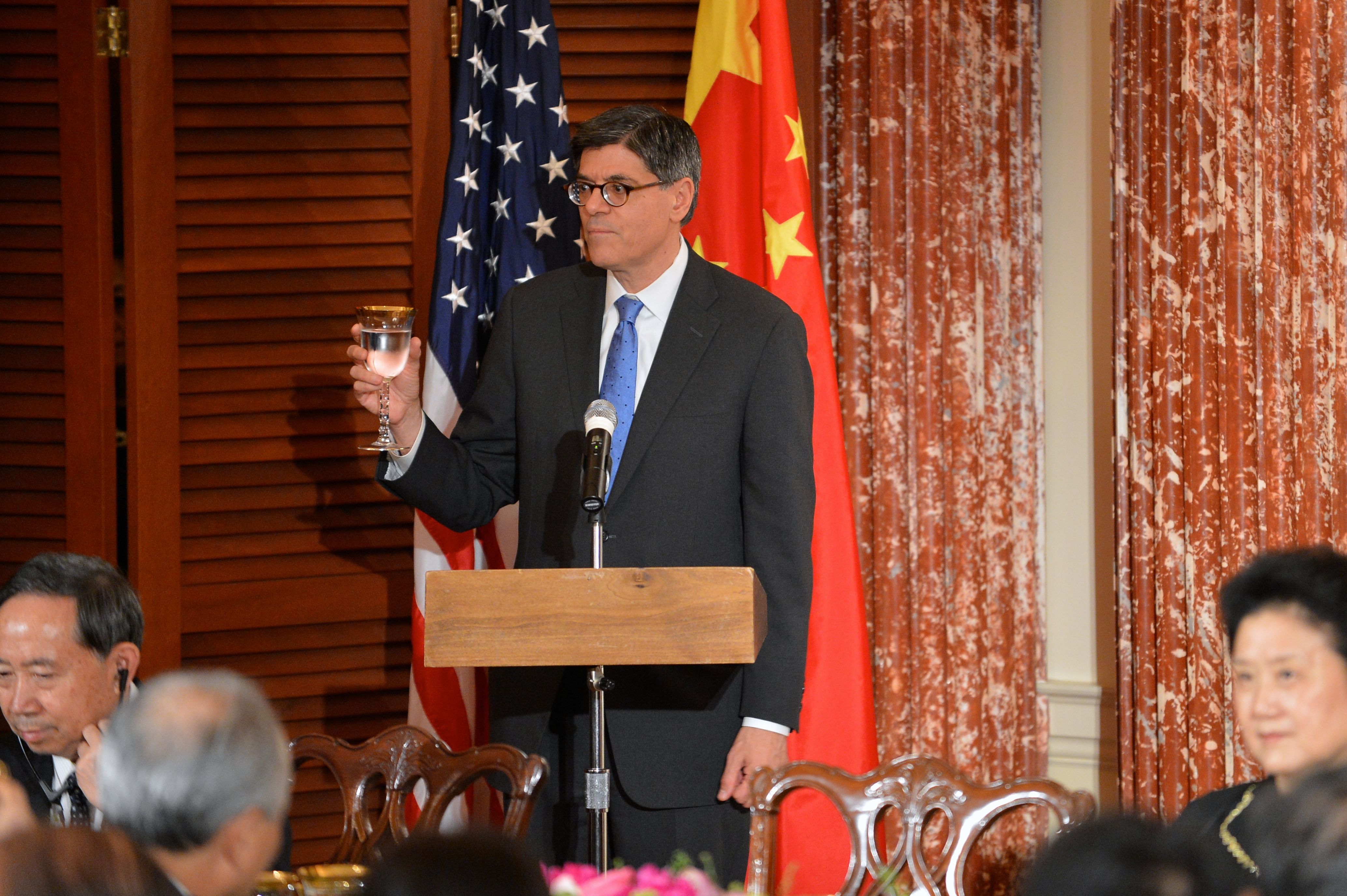The image depicts an indoor setting where a middle-aged man with greying black hair is standing at a wooden podium. He is dressed in a black suit with a white collared shirt and a light blue tie. He wears dark-framed glasses and has a serious expression. He is holding a glass with a bronze-colored stem containing a clear liquid, as if toasting the audience. 

The podium features a tall microphone positioned at the level of his tie. Behind him are two flags: an American flag on the left side of the image and a Chinese flag on the right. The background includes long, brown and yellow curtains beside wooden paneled doors or shutters.

In the foreground, several people are seated around a table, some facing towards the man and others facing away, indicating they are engaged in listening to a presentation.